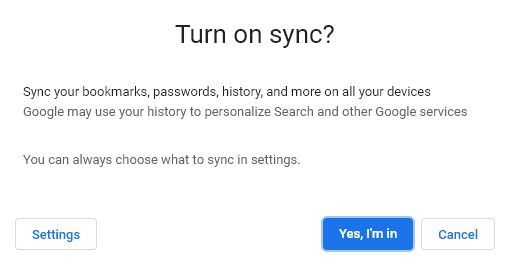The screenshot displays a user interface with a solid white background, which is landscape-oriented as it is slightly wider than it is tall. There is no border framing the image, giving it a clean and uncluttered presentation. The content suggests that the screenshot captures a portion of an application or settings menu.

At the top of the screen, centrally aligned in a larger font, the text reads "Turn on sync?", posing a question to the user. Directly beneath this heading, a smaller font explains the benefits of enabling sync: "Sync your bookmarks, passwords, history, and more on all your devices." This is followed by an additional note: "Google may use your history to personalize search and other Google services."

There is a gap before the next line, which is aligned to the left and mentions: "You can always choose what to sync in settings."

At the very bottom of the screen, three buttons are displayed. On the lower left, there is a blue button outlined in gray, labeled "Settings." On the lower right, there are two adjacent buttons. The first is filled with solid blue, indicating it is the currently selected option, and it reads "Yes, I'm in." Next to it, another button outlined in blue and labeled "Cancel" provides an opt-out option.